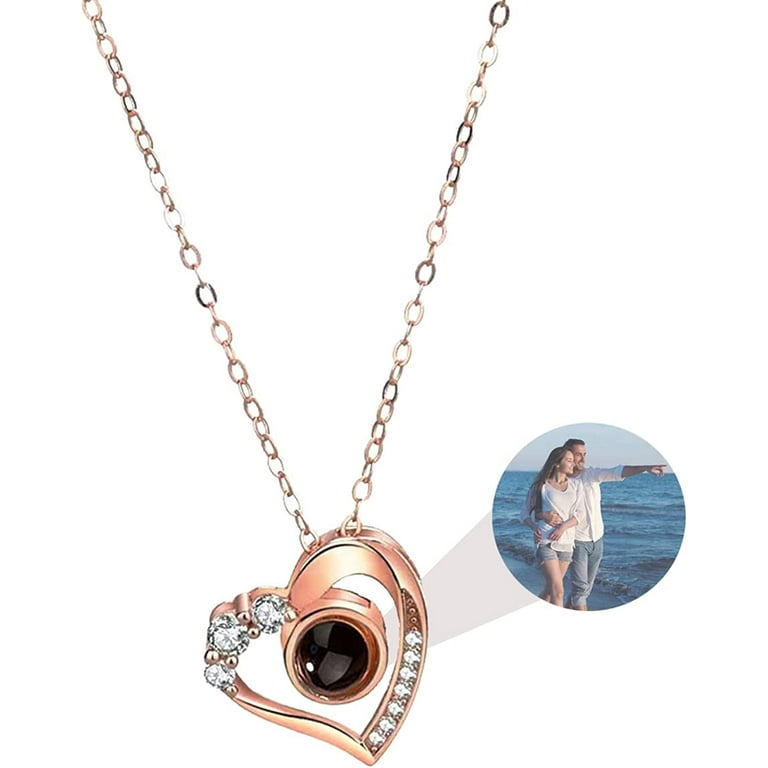The image showcases a heart-shaped pendant, crafted in rose gold and adorned with diamond-like stones. The left side of the heart features three large diamonds, while the right side is embellished with around seven smaller stones. At the center of the heart lies a striking dark stone, possibly black or dark brown onyx. This elegant pendant hangs from a rose gold chain. Adjacent to the pendant is a vivid image of a couple dressed in white shirts, with the woman wearing short jean shorts and the man in jean pants, walking along a beach. The man has his arm around the woman's waist as he points into the distance, capturing a serene and intimate moment by the water. This detailed and evocative presentation suggests the pendant symbolizes enduring romance and cherished memories.